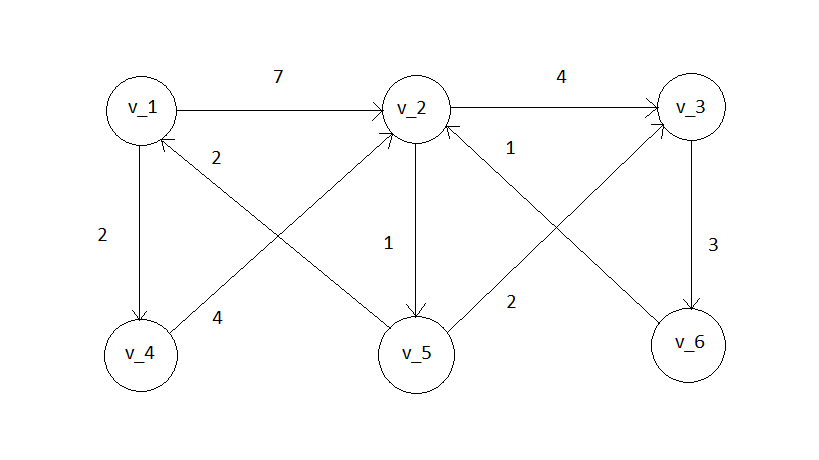This diagram features six labeled circles connected by directional arrows, each annotated with numerical values. The circles, labeled from V1 to V6, are positioned in the following layout:

- **Upper left:** Circle labeled V_1.
- **Right of V_1:** Circle labeled V_2, connected by an arrow from V_1 with a '7'.
- **Right of V_2:** Circle labeled V_3, connected by an arrow from V_2 with a '4'.
- **Bottom left, aligned horizontally:** Circles labeled V_4, V_5, and V_6 from left to right.
- **V_4:** Positioned directly below V_1, connected by an arrow from V_1 with a '2'.
- **V_5:** Positioned directly below V_2.
- **V_6:** Positioned directly below V_3.

Additional connections include:
- V_3 to V_6 with an arrow labeled '3'.
- V_6 to V_2 with an arrow labeled '1'.
- V_4 to V_2 with an arrow labeled '4'.
- V_2 to V_5 with an arrow labeled '1'.
- V_5 to both V_1 and V_3 with arrows labeled '2'.

The diagram forms open box-like shapes with intersecting connections, suggesting network or relational mappings, indicated by the placement of the arrows and their respective labels.